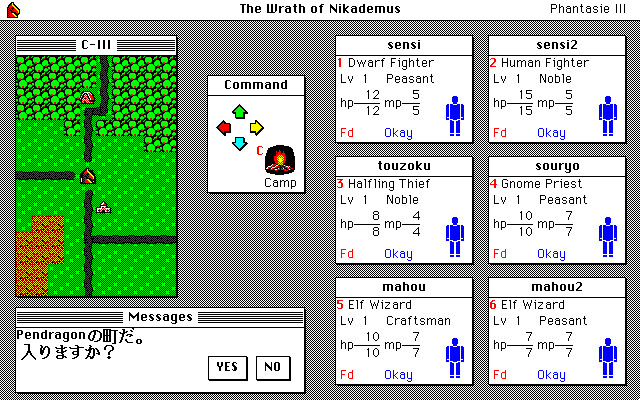This is a color screenshot from an early video game titled "Phantasie III: The Wrath of Nicodemus". The central playfield is rectangular with a gray background. On the upper left is a green field map depicting paths through woods and grass, showing locations like a cabin and a castle. The head of a brown knighted horse marks the player's location on the map. Below the map is a white message bar with "yes" or "no" options. 

Just above center and slightly left is a white "command" box with a directional pad featuring colored arrows: green (top), yellow (right), blue (bottom), and red (left). Adjacent to this on the right is a "camp" symbol with an icon of a campfire. Underneath this command interface is a vertically arranged set of blocks displaying character information. The characters listed are: 

1. Sensi (dwarf fighter) 
2. Sensi II (human fighter) 
3. Tozoku (halfling thief) 
4. Souryo (gnome priest) 
5. Mahou (elf wizard) 
6. Mahou II (elf wizard) 

Each block shows detailed information about the characters, including their speeds and abilities, complemented by blue silhouettes. At the top of the screen, the game title "The Wrath of Nicodemus" is centrally displayed, with "Phantasie III" in the top right. The overall scene combines elements typical of early video games, including a rudimentary map, command options, and character selection.